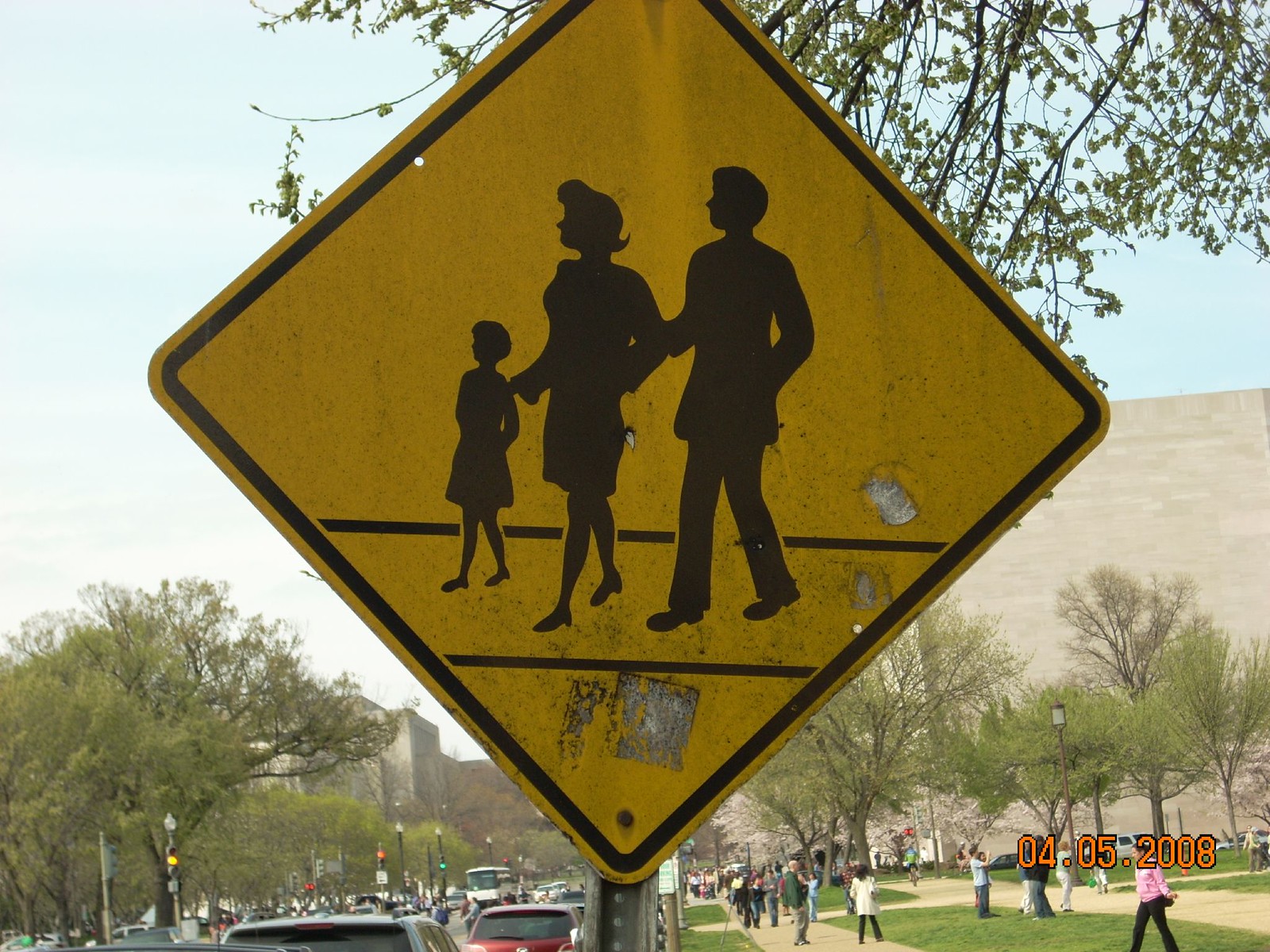This close-up photograph captures a diamond-shaped yellow street sign mounted on a gray metal pole. The sign, bordered in black, features the silhouette of a man, a woman, and a child holding hands as they traverse a crosswalk, depicted by two parallel black lines. The surface of the sign is notably dirty and bears remnants of previously affixed stickers or paper, now worn away and leaving behind a patchwork of residue.

In the background to the right, there is a bustling university campus. Students and pedestrians crowd the area, emphasizing the vibrant campus atmosphere. A prominent building, typical of collegiate architecture, dominates the background, while the adjacent road teems with vehicular traffic, highlighting the urban setting of the scene.